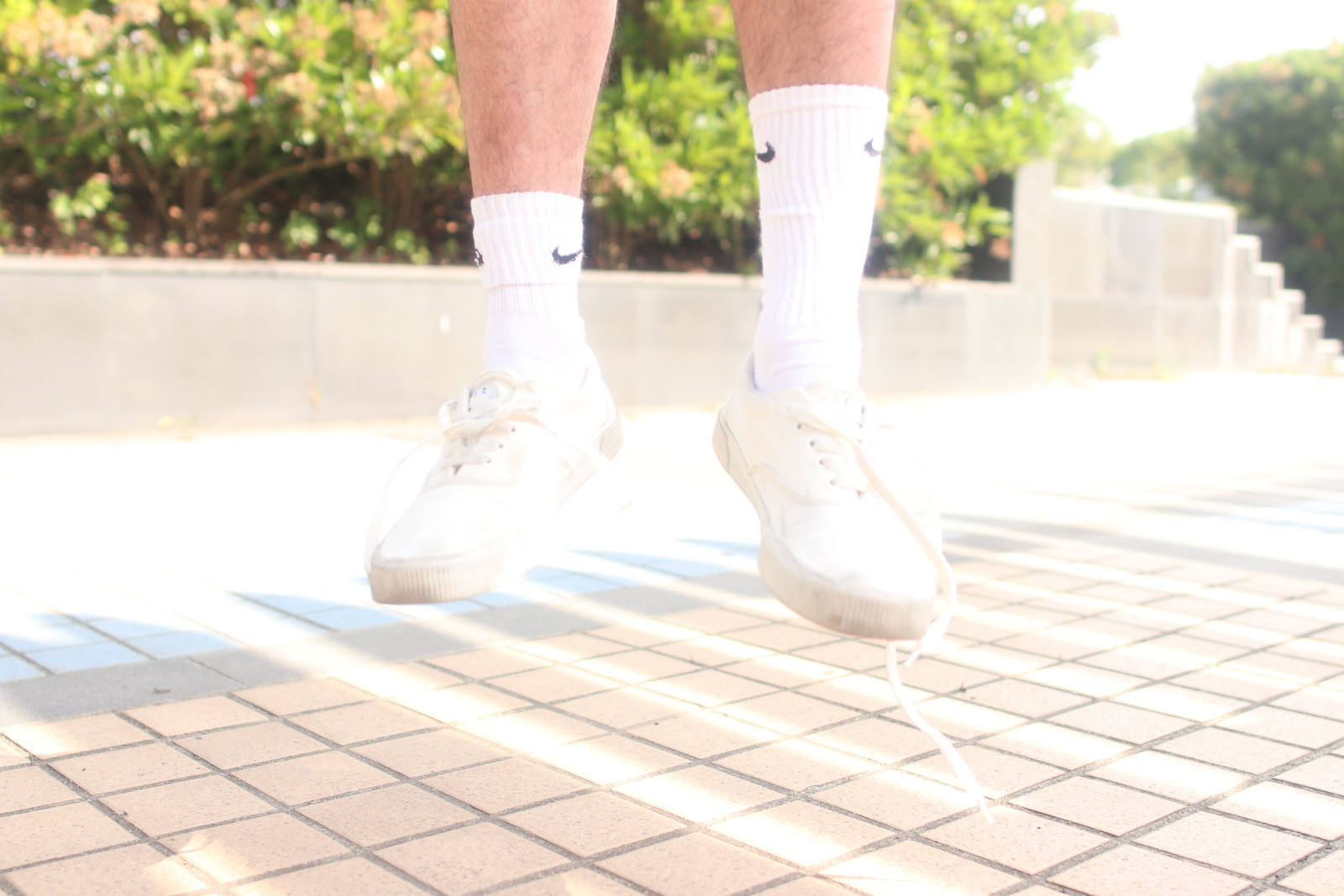In this color photograph with a landscape orientation, the focus is on a man's feet and lower legs as he jumps about a foot high off the ground on an outdoor beige square tile terrace. The man's bare legs, covered in dark hair, are shown in mid-air, cut off at the shins. He is wearing white, canvas lace-up sneakers, with the right shoelace untied and dangling beneath the shoe. His socks are white crew socks featuring the black Nike Swoosh logo; notably, the right sock is taller than the left. The scene’s backdrop includes a half stone wall in light gray, and behind the wall, there are dark green shrubs and bushes, indicating the outdoor setting. The photograph captures the moment in a style that blends photographic representationalism and video freeze-frame realism, with sunlight casting low light on the ground.